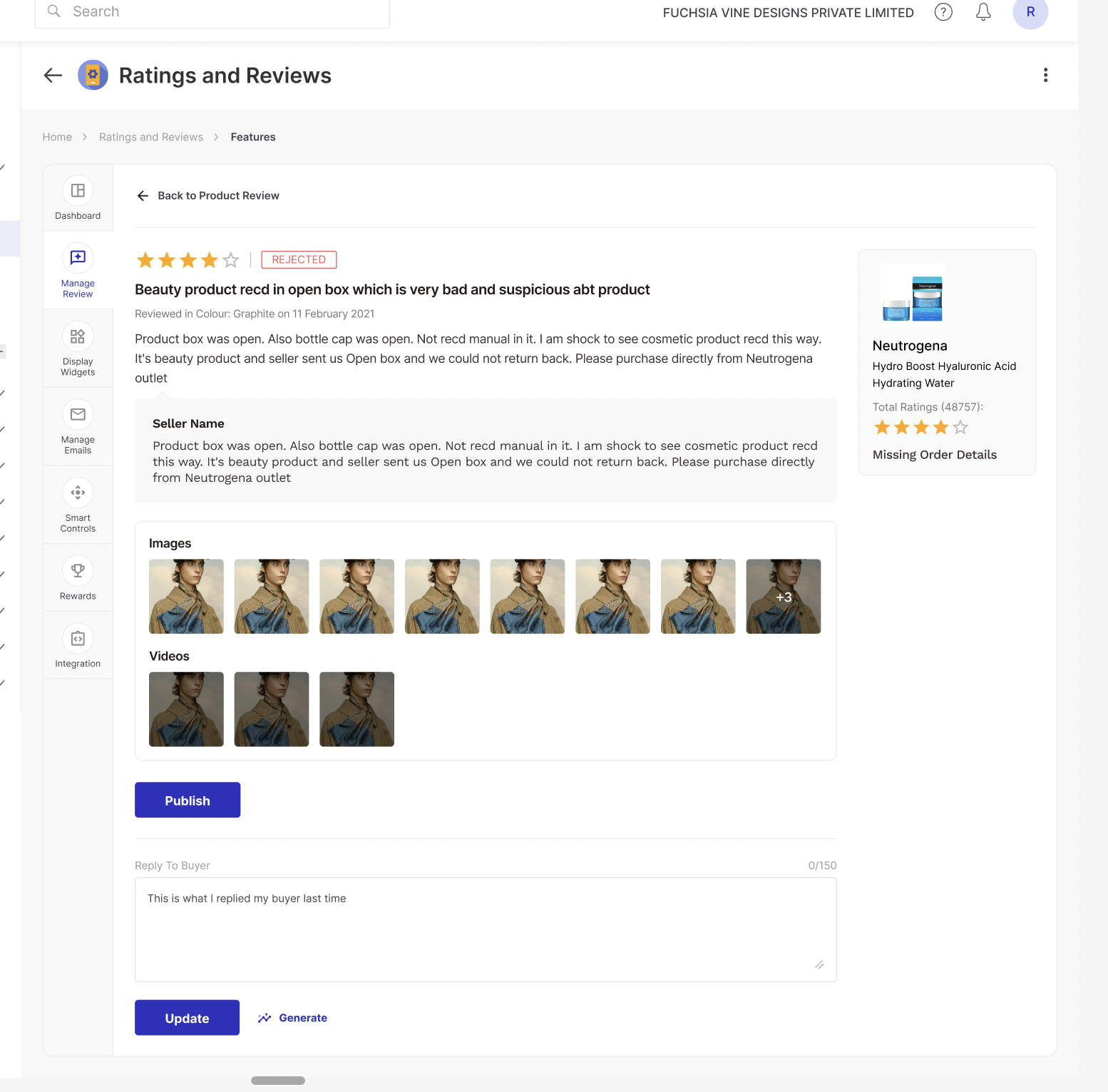The image showcases a screen capture from an e-commerce platform, possibly resembling eBay, where users rate and review products. The review in focus details a poor experience with a beauty product. Key points from the review include:

1. The product in discussion is "Neutrogena Hydro Boost Hyaluronic Acid Hydrating Water."
2. The reviewer received the product in an open box, with the bottle cap also open, and the manual missing, raising suspicions about its authenticity and safety.
3. Despite these issues, the product holds a 4 out of 5-star rating based on approximately 50,000 reviews.
4. The reviewer advises others to purchase directly from a Neutrogena outlet to avoid such problems.
5. The seller's name indicates awareness of the issue but lacks a resolution or return option.

The interface displays eight images and three videos, all essentially identical but gradually darkening, showing a girl wearing a dress. The text on the platform is primarily black and white, with yellow used for star ratings. The setup evokes a sense of familiarity with other retail sites where users can leave feedback and ratings on their purchases.